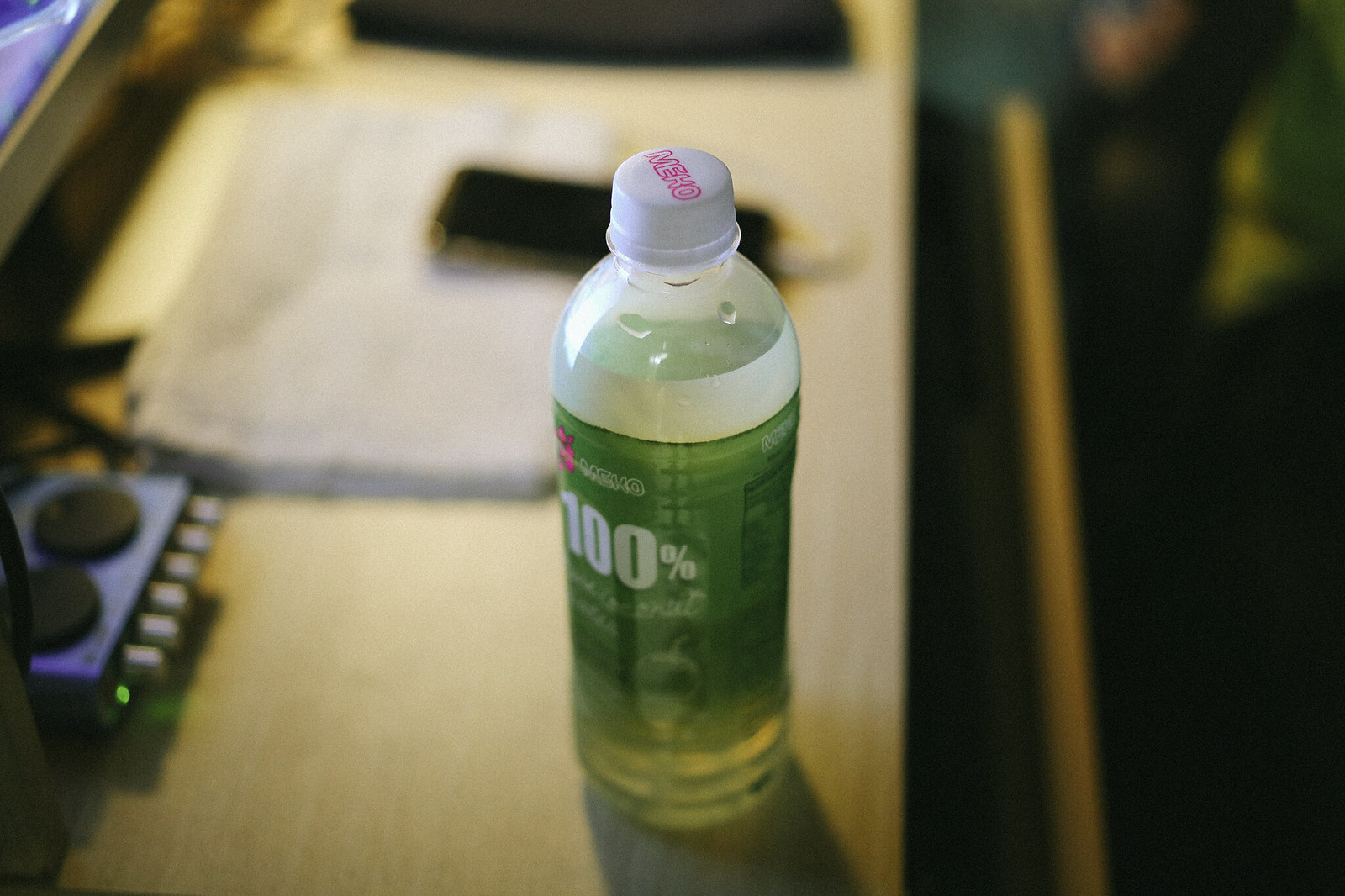The image features a highly detailed and sharply focused photograph of a bottle filled with a clear liquid, likely water. The perspective is a downward angle, presenting the bottle's white cap adorned with pink lettering at the top. The translucent body of the bottle showcases the liquid within, accentuated by a green label that dominates the lower portion. On the left side of the label, a pink flower is prominently displayed next to a brand name. Below this, "100%" is printed in bold white text, followed by a line of white cursive lettering. The reverse side of the label features small black text. The bottle rests on a light tan-colored table. In the background, there is a black phone and some electrical equipment with multiple gray knobs on the left side. The right side of the image is blurred, mostly black with a hint of green in the top-right corner.